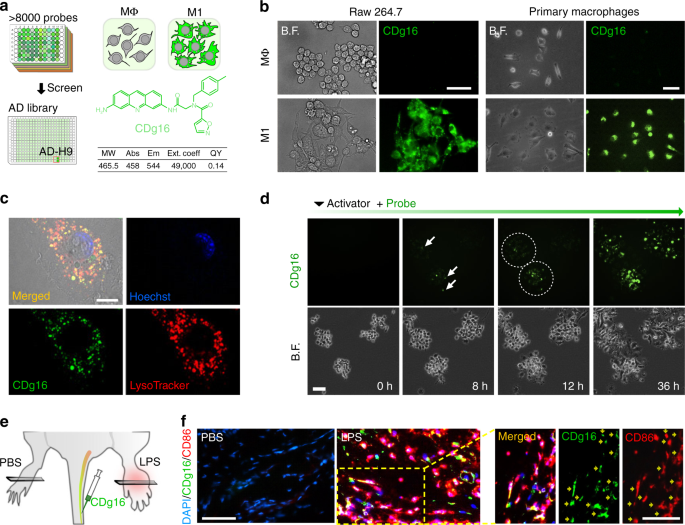The image displays an educational brochure or page from a kid's learning book, featuring various microscopic observations. It is divided into six distinct sections labeled A through F. Section A, on a white background, includes over 8,000 probes labeled 'M theta', 'M1', and an 'AD library', along with five boxes containing images resembling cells or spores with green hair-like structures. Section B, also showing a white background, displays raw data labeled '26.7' and images of cells. Sections C and D, set against black backgrounds, each feature multiple sub-boxes with microscopic images of cells, with section C's top left box merged, the top right bordered in blue, and the bottom left labeled 'CDG16'. Section E, on a white background, depicts what appears to be the lower half of an amphibian. Finally, section F shows colorful microscopic cells. The overall color palette includes shades of gray, green, black, red, and pink.